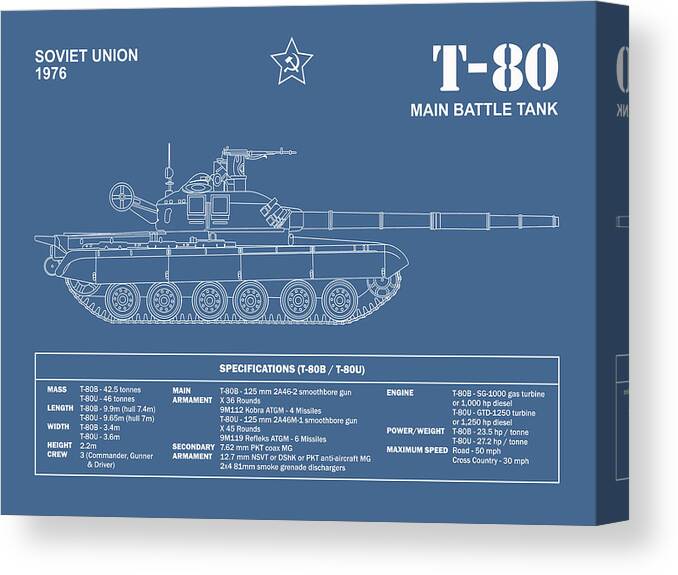The image depicts a rich blue canvas that showcases a detailed diagram of the Soviet Union's T-80 main battle tank. The tank is illustrated in white lines, with its cannon facing towards the right. At the top left corner, the text "Soviet Union 1976" is printed, accompanied by the Soviet Union emblem, a white hammer and sickle inside a star. On the top right, bold white letters spell out "T-80 Main Battle Tank." Below the tank illustration, a rectangular box labeled "Specifications" lists detailed information about the tank's mass, length, width, height, crew composition, engine power, weight, and maximum speed. The overall design appears digitally animated, emphasizing the contrast of the white outline and text against the blue background.